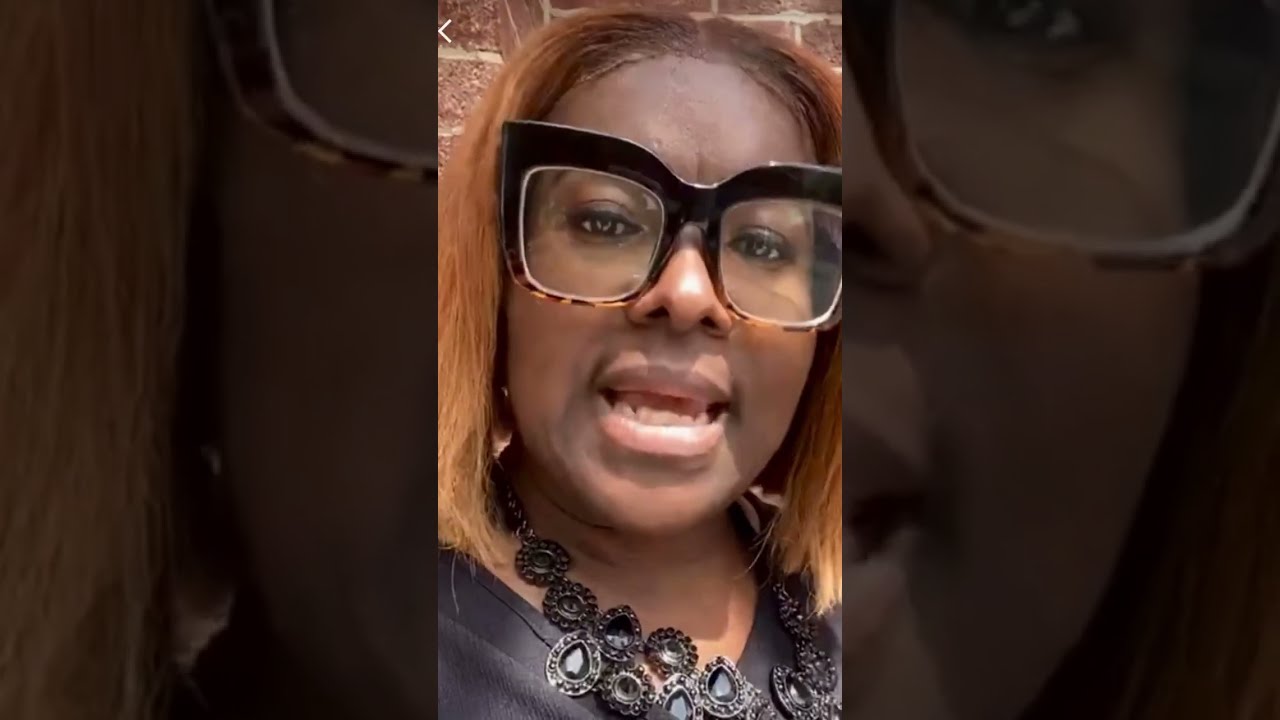This image captures an African American woman with dyed reddish-brown hair, styled down. She is wearing distinctive eyeglasses with thick black frames at the top and a tortoise shell design at the bottom. Her mouth is open as though she is speaking. She accessorizes with a large, ornate black necklace featuring black gemstones, and she is dressed in a black shirt. The background consists of a red brick wall with visible cement grout lines, suggesting she is outdoors, possibly in the sunlight.